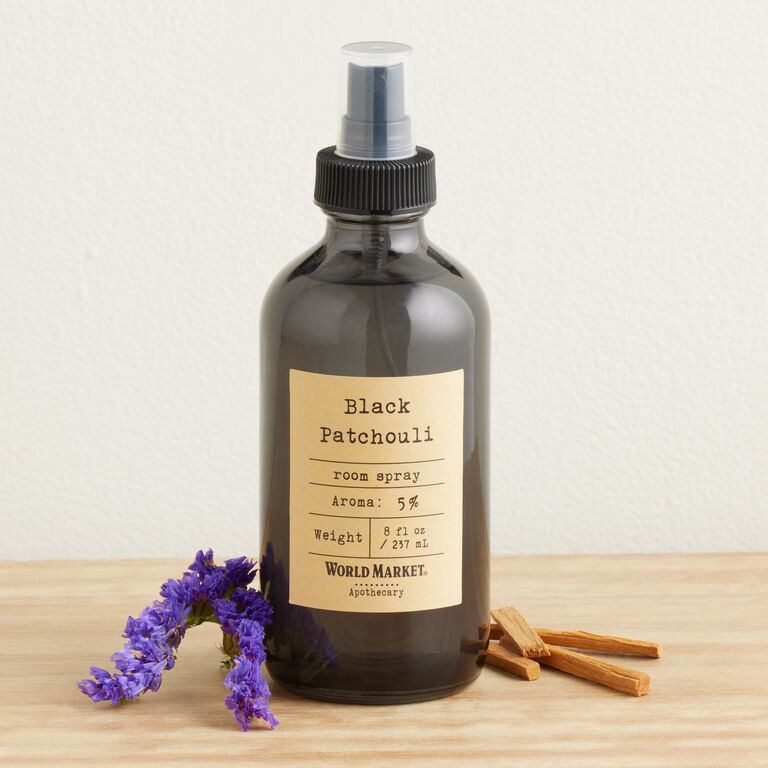The photograph features a central, vertically-aligned rectangular image of a brown glass bottle of room spray placed on a light-colored wooden surface. The background consists of a textured white wall. The bottle has a brown screw-type lid with a spray mist attachment, covered by a small clear cap. The label on the bottle is tan, stylized to mimic an old typewriter font. It reads "Black Patchouli," followed by a line, then "Room Spray," "Aroma 5%," "Weight 8 fluid ounces / 257 ml," and at the bottom, "World Market Apothecary," all centered in black font. The bottle is surrounded by small, broken pieces of wood to the right and sprigs of lavender flowers, which are purple, to the left.